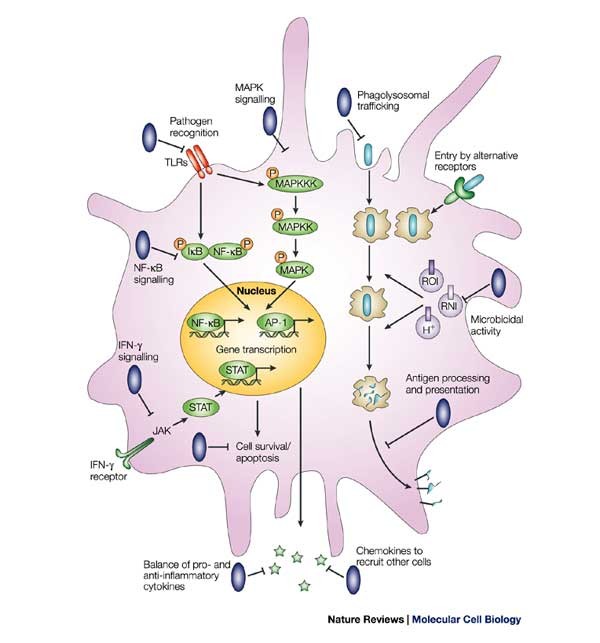The infographic from **Nature Reviews Molecular Cell Biology** features a detailed illustration of a cell on a white background with a light purple splatter effect and a thin black outline. The central focus of the infographic is the labeled components of a cell, including the nucleus prominently highlighted in yellow. 

In the top left corner, the diagram details "Pathogen Recognition" with labels for TLRs, highlighting where these receptors are located within the cell. Adjacent areas depict "MAPK Signaling" and "Phagolysosomal Trafficking," providing visual paths for these cellular processes with numerous bluish ovals.

To the upper right, the graphic shows "Entry by Alternative Receptors," illustrating various entrance points within the cell. Green ovals with clockwise arrows are labeled as "Gene Transcription," indicating areas of genetic processing. 

Additional elements are marked throughout the cell, including "Cell Survival," "Apoptosis," "Antigen Processing and Presentation," and "Microbicidal Activity," offering a comprehensive overview with intricate labeling and connections. Each section is linked by black lines and arrows, further clarifying the complex cellular interactions.

Overall, this infographic serves as an intricate and detailed resource on cellular structure and function, emphasizing the interconnected processes critical for cell biology.